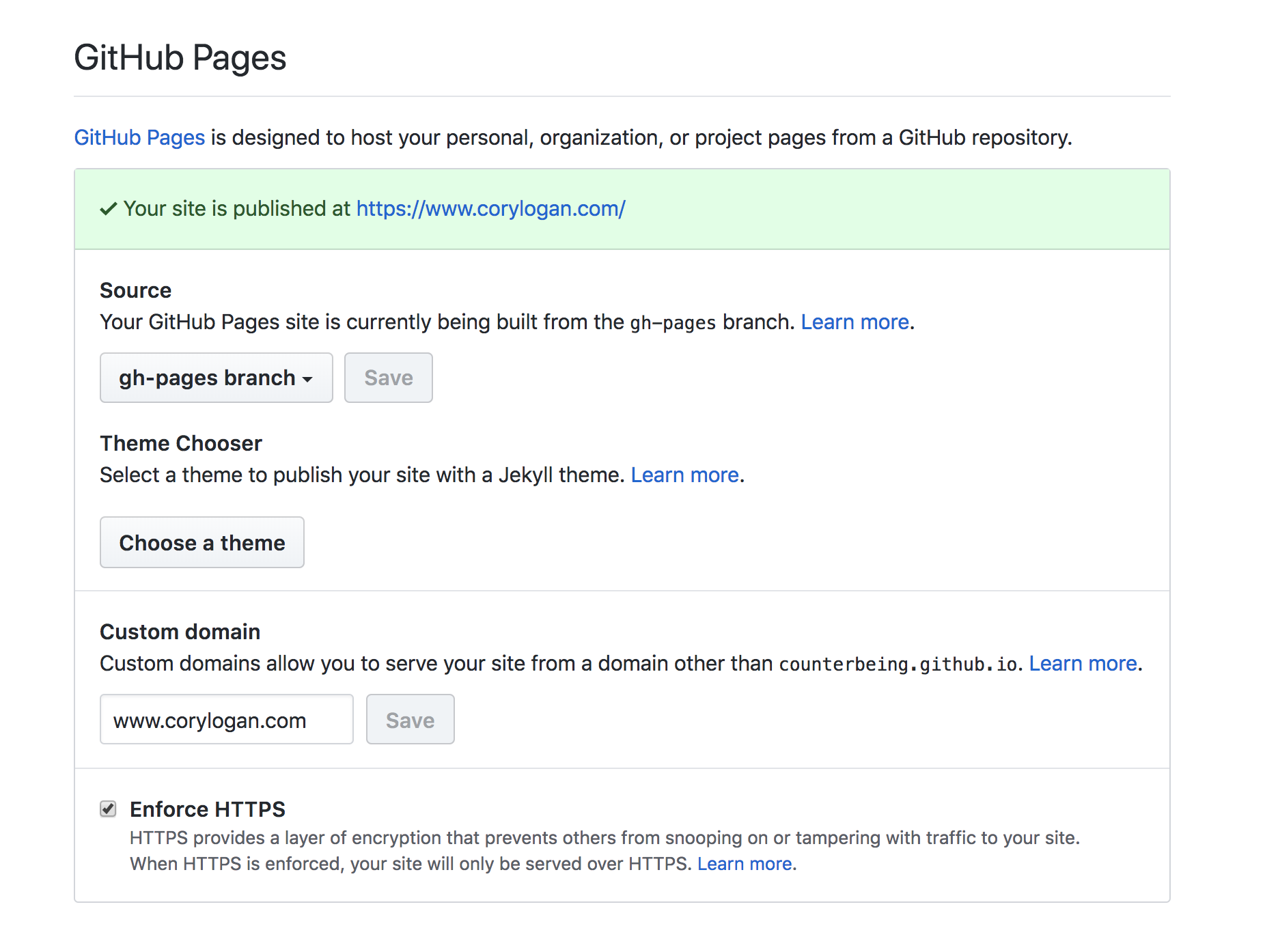This screenshot from GitHub showcases the settings for a GitHub Pages site, specifically from the repository associated with the user or organization "counterbeing." At the top of the interface, the title "GitHub Pages" is prominently displayed. This feature allows users to host personal, organizational, or project pages directly from a GitHub repository.

The site in question is published at the URL: [https://www.corylogan.com/](https://www.corylogan.com/). It is noted that the GitHub Pages site is built from the "gh-pages" branch of the repository, with an option to "Learn more" for additional details.

Under the "Theme chooser" section, users are prompted to select a Jekyll theme to style their site, with a link to "Learn more" about the available themes. Custom domain settings specify that sites can be served from domains other than the default "counterbeing.github.io." The current custom domain in use is "www.corylogan.com."

There is an option to "Enforce HTTPS," which has been checked. This ensures that the site is served securely over HTTPS, providing encryption to prevent unauthorized access or tampering with site traffic. Again, a "Learn more" link is provided for further information on HTTPS.

The image does not include any people.